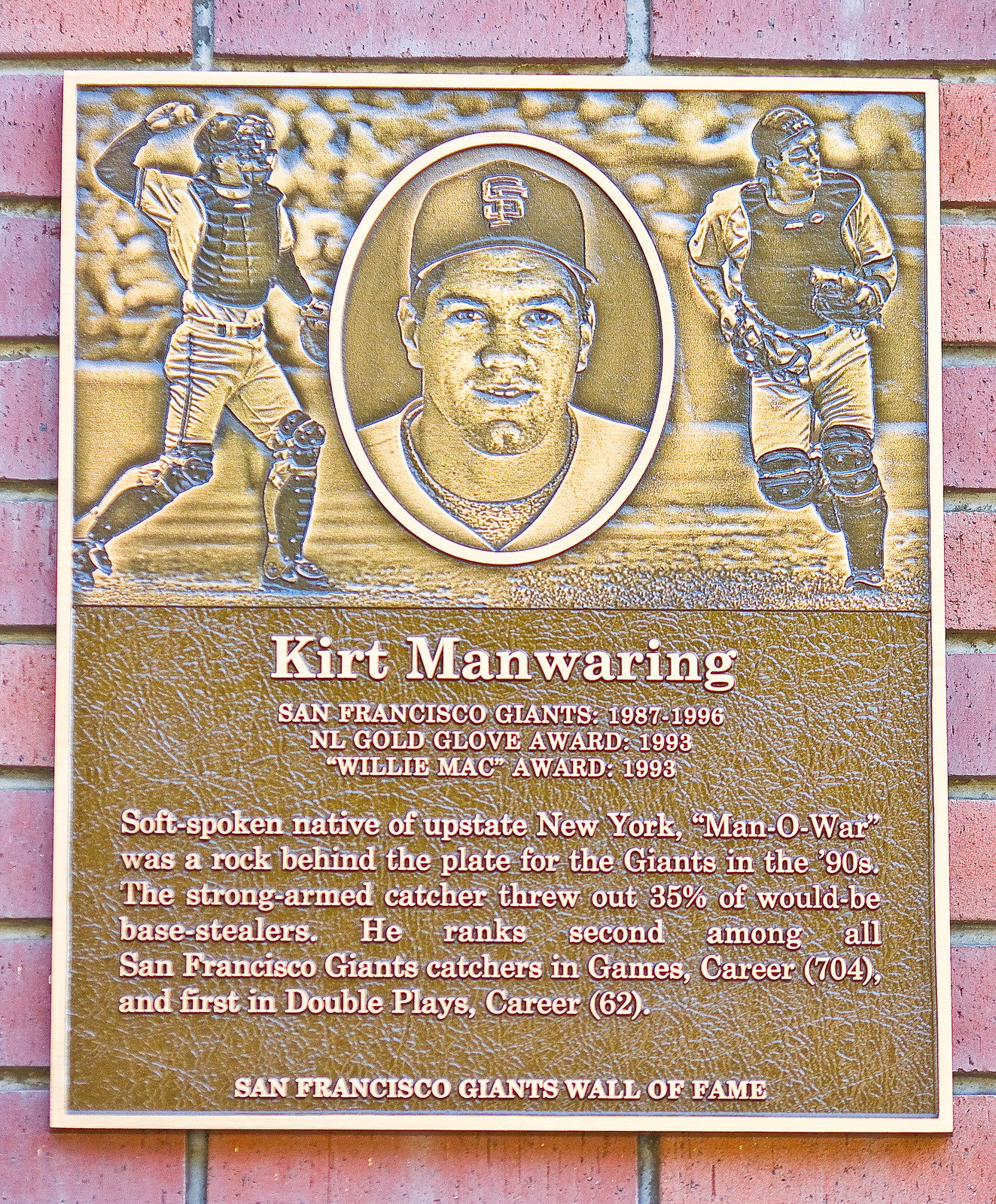The plaque on the red brick wall commemorates Kurt Manwaring, who played for the San Francisco Giants from 1987 to 1996. The square plaque, featuring a mix of bronze, black, and white colors, includes a main central image of Manwaring, a white male player, wearing a black cap with the SF logo for the San Francisco Giants and a white uniform. This primary image is flanked by two action shots: on the left, Manwaring is throwing a ball while wearing a black catcher's vest; on the right, he is running, also in his catcher's gear. 

The text below the images reads: "Kurt Manwaring, San Francisco Giants 1987-1996, NL Gold Glove Award 1993, Willie Mack Award 1993." Further down, it provides a description: "A soft-spoken native of upstate New York, 'Man O' War' was a rock behind the plate for the Giants in the 90s. The strong-armed catcher threw out 35% of would-be base stealers. He ranked second among all San Francisco Giants catchers in games played (704) and first in career double plays (62). San Francisco Giants Wall of Fame." This detailed plaque celebrates Manwaring's significant contributions to the team and his impressive defensive skills.